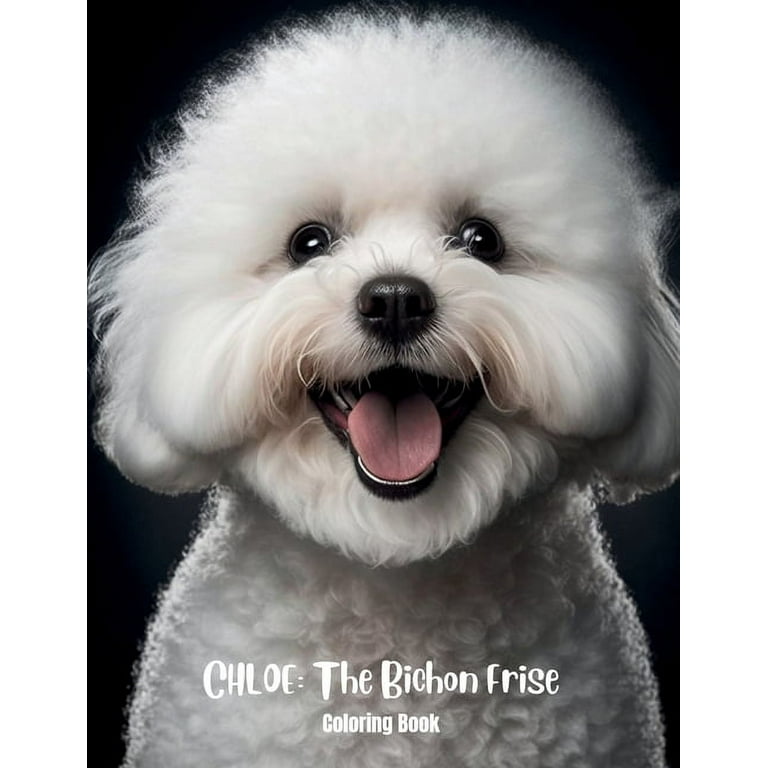The front cover of the "Chloe, the Bichon Frise Coloring Book" features an actual photograph of a white Bichon Frise dog with fluffy, tight curly hair. The dog's mouth is open, as if smiling, revealing a pink tongue and black bottom lip. The white fur is especially prominent against the solid black background, which also highlights the black nose and eyes, the latter buried in the fluffy hair. Light gleams off the hair on both sides of the dog's head, adding depth to the close-up image that captures part of its torso and head, with the ears hidden in the fluffiness. The title "Chloe, the Bichon Frise Coloring Book" is printed in white letters at the bottom of the cover.